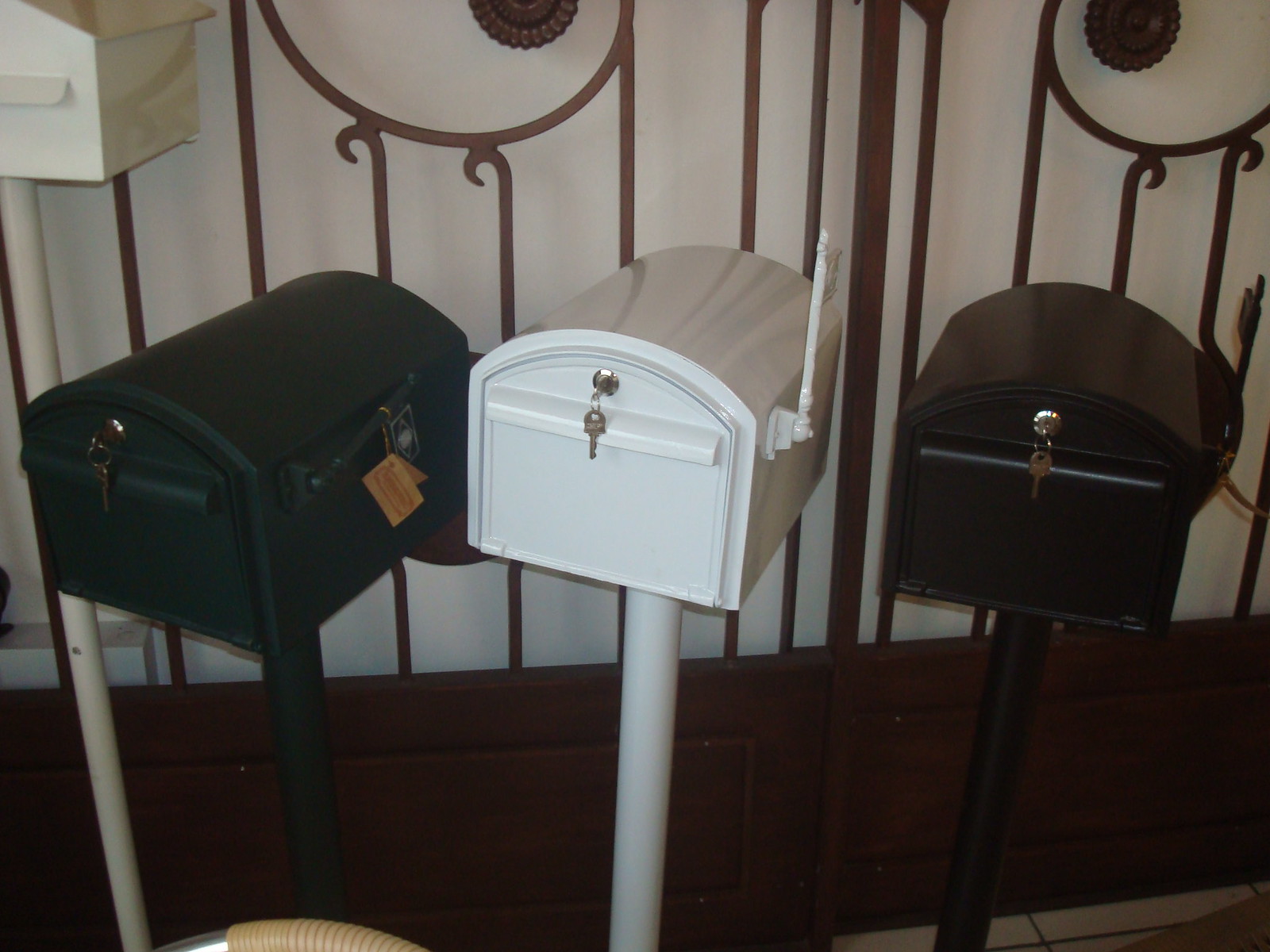The image captures a close-up of three mailboxes on display, possibly in a store. Each mailbox is mounted on a metal pole, corresponding in color to the mailbox itself. The mailbox on the left is a dark navy green, the one in the center is white with its red flag raised, and the one on the right is black. All mailboxes feature arched roofs and have locks with keys hanging out, indicating they are lockable. The background includes intricate metal fencing leaning against a white wall, suggesting an outdoor theme within this indoor setting. The floor appears to be white-tiled, and at the bottom of the frame, part of a chair is visible. The overall scene is dimly lit, enhancing the detailed textures of the mailboxes and their surroundings, while no text is present in the image.